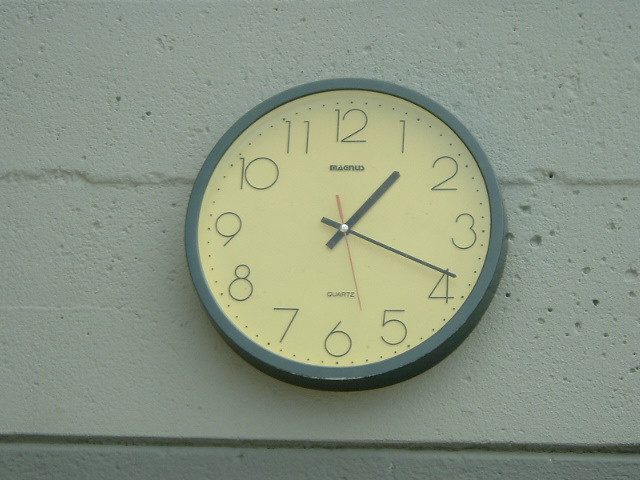This image showcases an analog clock mounted on a textured wall. The clock features a dark blue plastic frame with a yellow face inside, contrasting sharply with its thin, dark blue numerals. Three hands—a minute hand, an hour hand, and a red second hand—are centrally anchored by a silver pin. At the top of the clock face, black text spells out "MAGNUS," and at the bottom, the word "QUARTZ" is similarly written in black. The surrounding wall, reminiscent of concrete with sponge-like recesses and slight cracks, is of a pale grayish or off-white hue, suggesting an environment like an office, a classroom, or a governmental building. The clock is centered within the frame of the image, drawing immediate focus.